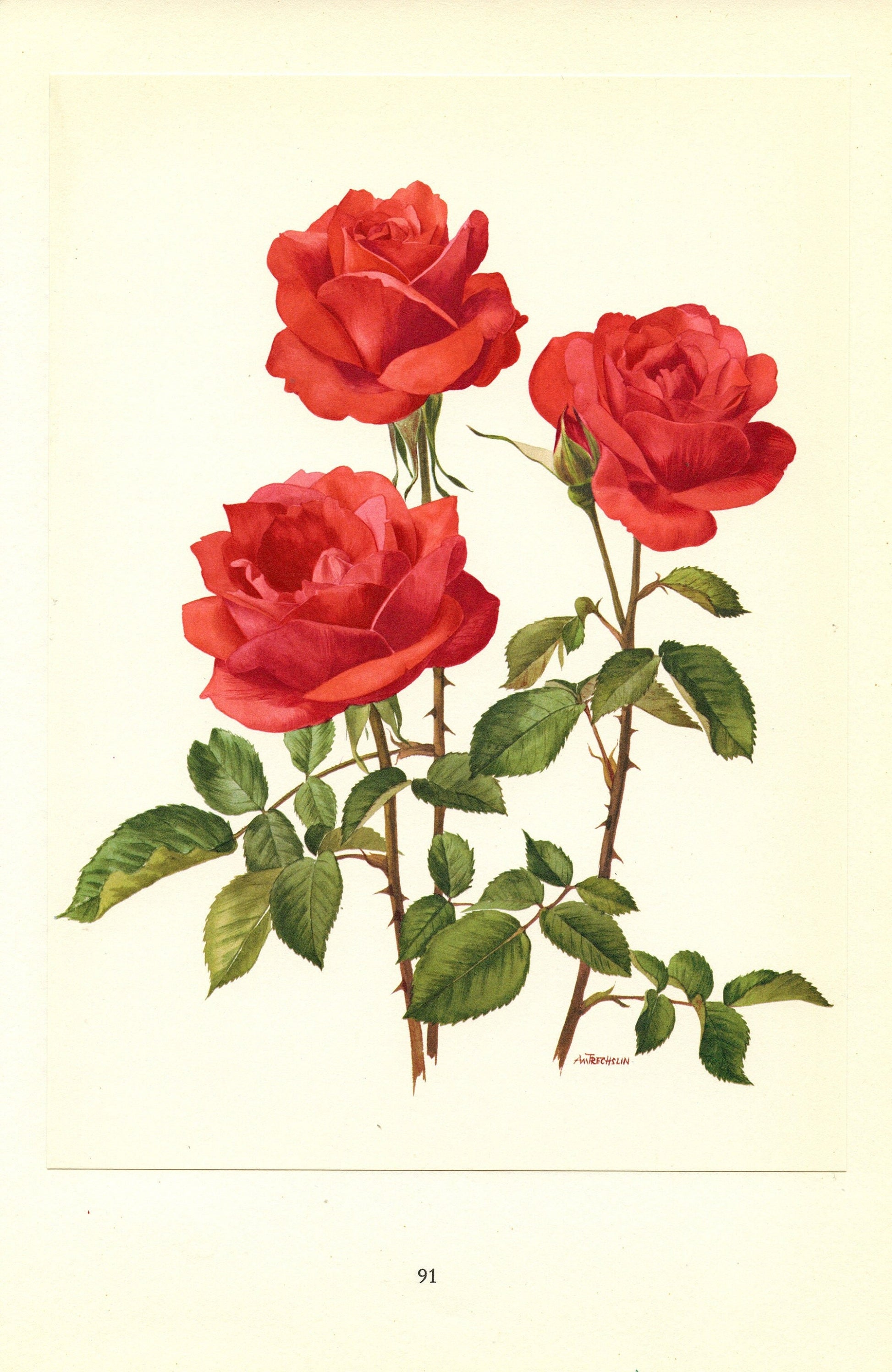This is a highly detailed illustration, likely from a book, depicting three red roses with intricate line work. The roses vary in shape but are similar in size, with the one on the right being the tallest and featuring an unbloomed rose bud offshooting to the left. Each rose exhibits brown stems adorned with thorns and serrated green leaves, meticulously rendered to showcase their natural beauty. The artwork sits on a cream-colored background within a tall rectangular frame, suggesting it may be a book page, supported by the presence of a small black "91" at the bottom, resembling a page number. Additionally, there is a thin line above the number, possibly a page divider, and an indistinct watermark reading "Lin..." at the lower edge.